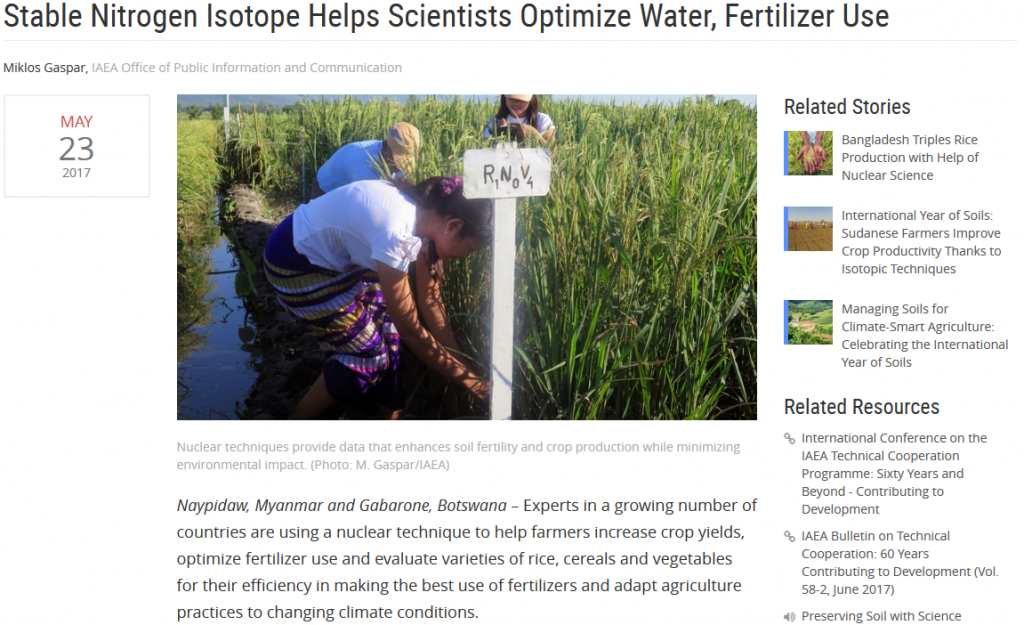**Caption:**

"Stable Nitrogen Isotope Helps Scientists Optimize Water Fertilizer Use" by Miklos Gaspar, dated May 23, 2017.

The composite image features two juxtaposed scenes. On the left, workers are seen laboring in verdant rice paddies, the fields visibly submerged in water. A conspicuous white sign, marked with "R1N0V4," stands amidst the lush growth. The right side of the image depicts a densely grass-covered area. 

Subtext:
Experts in a growing number of countries are utilizing a nuclear technique to assist farmers in boosting crop yields, optimizing fertilizer use, and evaluating various strains of rice, cereals, and vegetables. This method aims to enhance fertilizer efficiency and adapt agricultural practices to evolving climate conditions. Related stories and resources are listed on the right.